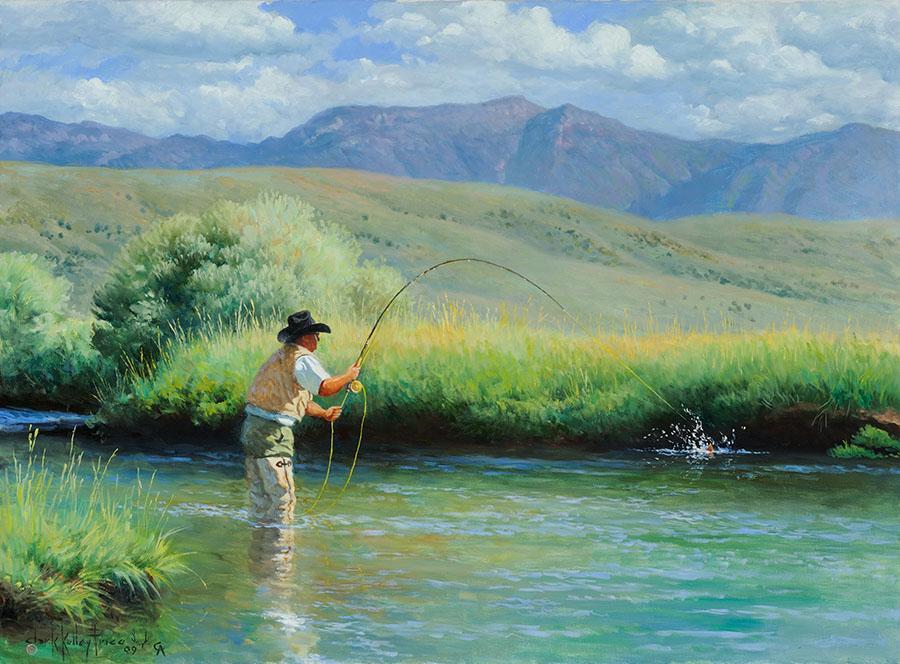This hyper-realistic painting depicts an outdoor scene centered around a man fly fishing in a river. The fisherman, located in the left center of the painting, is equipped with a black Stetson cowboy hat, a white shirt, a light brown fishing vest, and khaki-colored waders up to his thighs. He's holding a curved fly fishing rod, and you can see water splashing near the end of his line, suggesting he has hooked a fish.

The foreground features a tranquil river with various shades of blue and green, accented with white to capture the movement of water. To the bottom left, there is a cluster of green wreaths and tall grasses. Just behind the fisherman, a brush line composed of bushes and shrubbery transitions into a sprawling meadow with yellow accents, possibly indicative of wheat or flower fields.

The landscape extends into rolling hills of various shades of green that gently slope and merge into the horizon. Beyond the meadow and hills, large, majestic mountains rise, painted in hues of purple, brown, and gray. The sky overhead is dramatic and filled with fluffy white clouds, tinged with blue and hints of black, lending depth and contrast to the scene. The hyper-realistic details, despite visible brush strokes in the clouds, affirm the painting's professional craftsmanship. Additionally, a signature in black paint can be seen in the lower left-hand corner of the artwork.